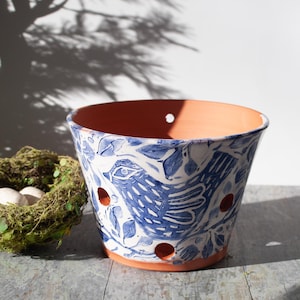This detailed photograph, taken outside on a sunny day, features a beautifully crafted terracotta flowerpot and a bird's nest side by side, set atop a grey marbled tile floor. Dominating the right half of the image, the flowerpot has an unpainted, earthy brownish-red interior, characteristic of traditional clay. In contrast, the exterior of the pot has been artistically painted with a white background and intricate blue designs—including leaves, floral patterns, and a central motif of a bird with a small beak, white stripes down its body, and partially visible wings. Notably, the pot features three holes: one near the bottom and two about halfway up. To the left of the flowerpot, the bird's nest, woven with brown and green materials, cradles two small white eggs. The bright sunlight casts a sharp shadow of a nearby tree onto the smooth, white background wall, adding depth and a natural touch to the scene. The cast shadow of the clay pot is also visible on the tiled surface, enhancing the outdoor ambiance of this captured moment.